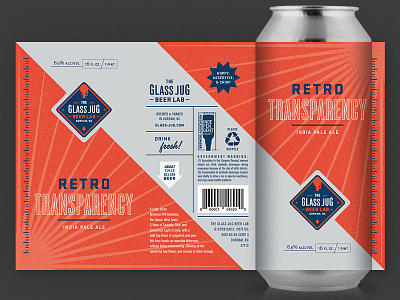This image features an advertisement for a beverage by The Glass Jug Beer Lab, prominently showcasing a single can of beer. The can, labeled as "Retro Transparency India Pale Ale," sports a vibrant palette of orange, silver, blue, white, and red colors. Positioned perpendicularly, the can appears to float against a stark black background, adding to the striking visual appeal. Notably, the label includes a barcode and a recycling symbol, emphasizing both the product and its packaging. The label appears to be peeled off and extended horizontally, providing a comprehensive view of all the design elements and text, which includes the tagline "Drink Fresh." The overall setting is purposefully minimalistic to keep the focus entirely on the can and its retro-themed design.